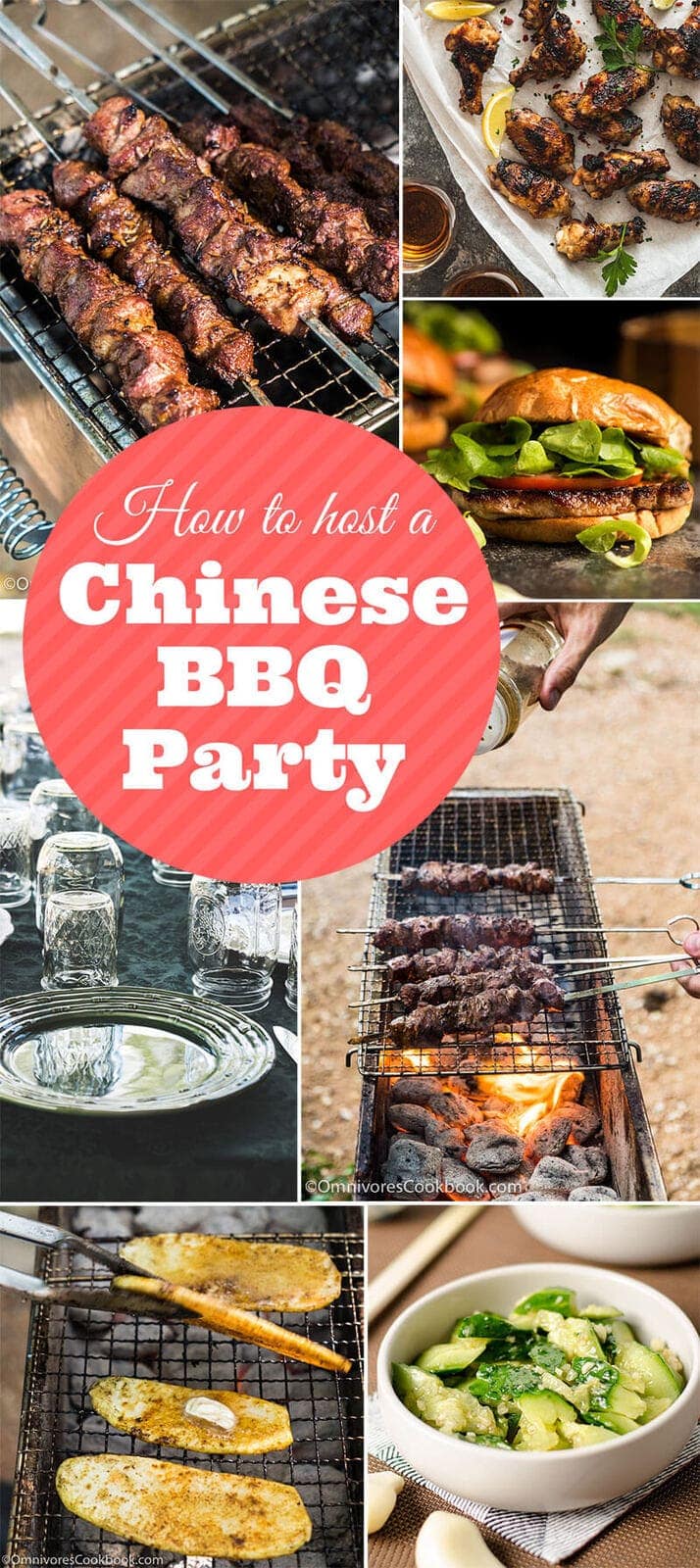This image is a vibrant and diverse collage illustrating how to host a Chinese barbecue party. At the center of the collage, slightly oriented to the right, is a prominent red circle with white text that reads, "How to Host a Chinese Barbecue Party." Surrounding this central text are seven distinct photographs, each showcasing various elements of the barbecue experience. 

One image captures skewers of meat sizzling on a grill, while another displays chicken wings and drumsticks artfully arranged on a white platter, garnished with lemon wedges and green herbs. A juicy hamburger with a visible patty, slice of tomato, and greens sticking out from the bun features prominently in one photograph.

Additional images include more meat skewers, one of which shows a hand sprinkling spices onto the meat, adding a touch of culinary action. Another image depicts utensils, plates, and mason jar-style tumblers, all set on a table ready for dining. There’s also a photograph of what appears to be a type of bread or grilled vegetable being flipped with tongs. Lastly, a bowl of diced green vegetables, possibly garnished with garlic, contributes a fresh contrast to the array of grilled dishes. 

A watermark in one of the photos, which repeats in the bottom left of the collage, credits omnivorescookbook.com. The rich details and vibrant food imagery combined with the central instructional text make this collage a comprehensive guide to hosting a Chinese barbecue party.